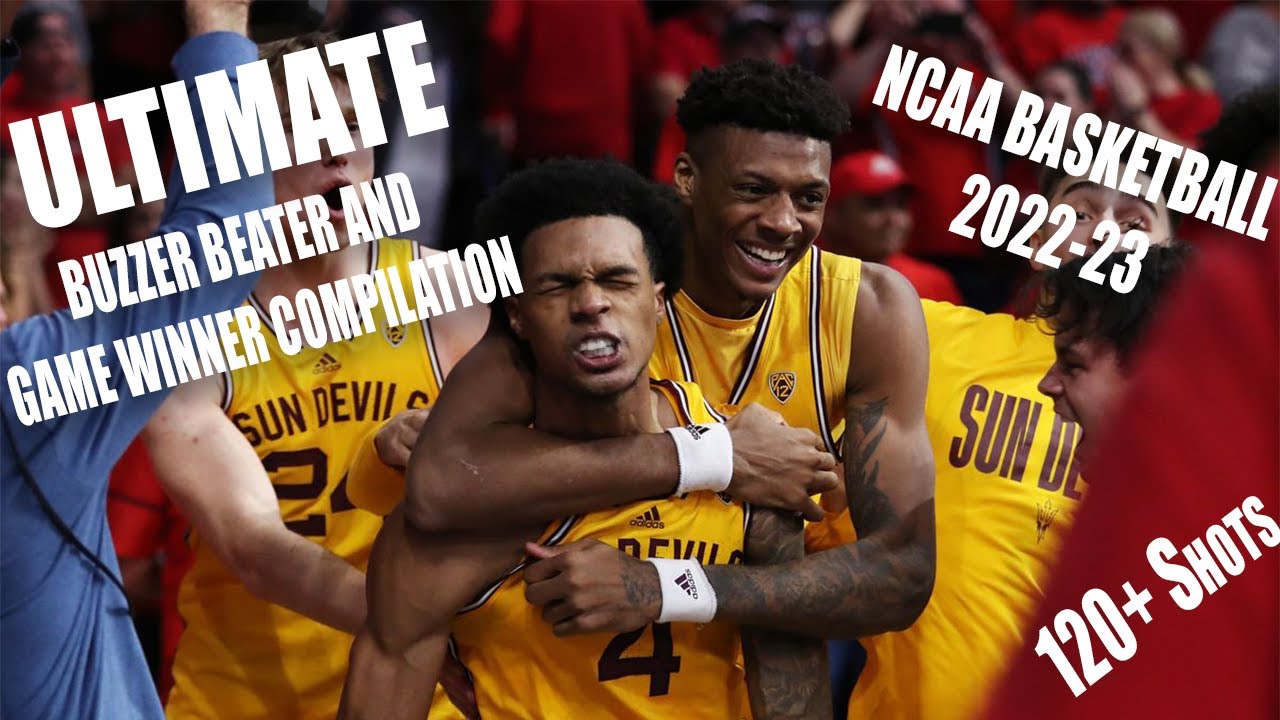This is a color photograph in landscape orientation featuring an emotional indoor scene from a basketball game. Central to the image are two African-American players in yellow jerseys, celebrating a victory. The taller player, donning white wristbands with markings, is hugging the smaller player from behind, who wears the number 4 on his jersey. Both appear exasperated yet jubilant, embodying the thrill of triumph. To the left of the embracing duo stands a white player in a jersey labeled "Sun Devils 24," while to the right, another white player faces away in a jersey partially visible with "Sun D" written on it. The top left corner of the image is overlaid with the text "Ultimate Buzzer Beater and Game Winner Compilation," while the top right corner features "NCAA Basketball 2022-23." In the bottom right corner, the text "120 plus shots" is displayed. The bottom left corner includes an inset of a white man in a blue long-sleeve shirt. Blurred red-clad figures can be seen in the background, adding to the atmospheric depth of the photograph. Likely serving as a YouTube video thumbnail, this captivating image combines realism with dynamic graphic design elements.